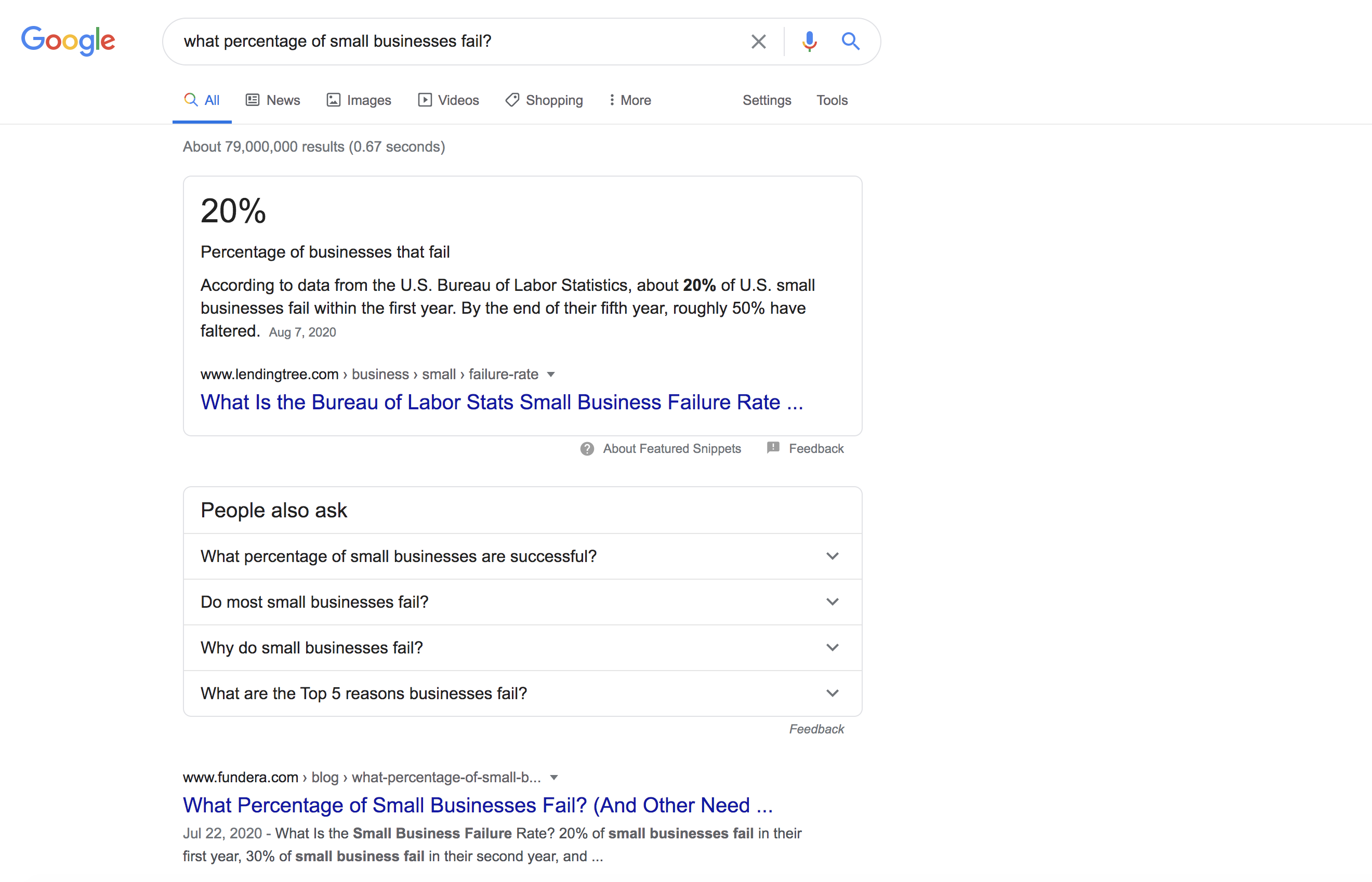The image is a screenshot of Google search results displaying information about the failure rates of small businesses. At the top, the Google logo is prominently displayed, followed to the right by the search bar, an "X" icon, a microphone icon, and a magnifying glass icon. The search query entered is "what percentage of small businesses fail," yielding approximately 79 million results in 0.67 seconds. The search is categorized under "All," as opposed to "News," "Images," "Videos," "Shopping," etc.

The top result indicates that, according to data from the US Bureau of Labor Statistics, about 20% of US small businesses fail within their first year. By the end of their fifth year, roughly 50% have faltered. This information comes from an article dated August 7, 2020, on LendingTree.com. Below this result is a blue hyperlink asking, "What's the Bureau of Labor stats for small business failure rate?"

Further down, the "People also ask" section lists related questions such as "What percentage of small businesses are successful?", "Do most small businesses fail?", "Why do small businesses fail?", and "What are the top five reasons businesses fail?" Another link from fundera.com (partially cut off in the screenshot) addresses "What percentage of small businesses fail and other ..." providing further insights into business failure rates.

Overall, the screenshot serves as a summary of publicly available data from the Bureau of Labor Statistics, capturing key statistics about small business survival rates within the first five years of operation.